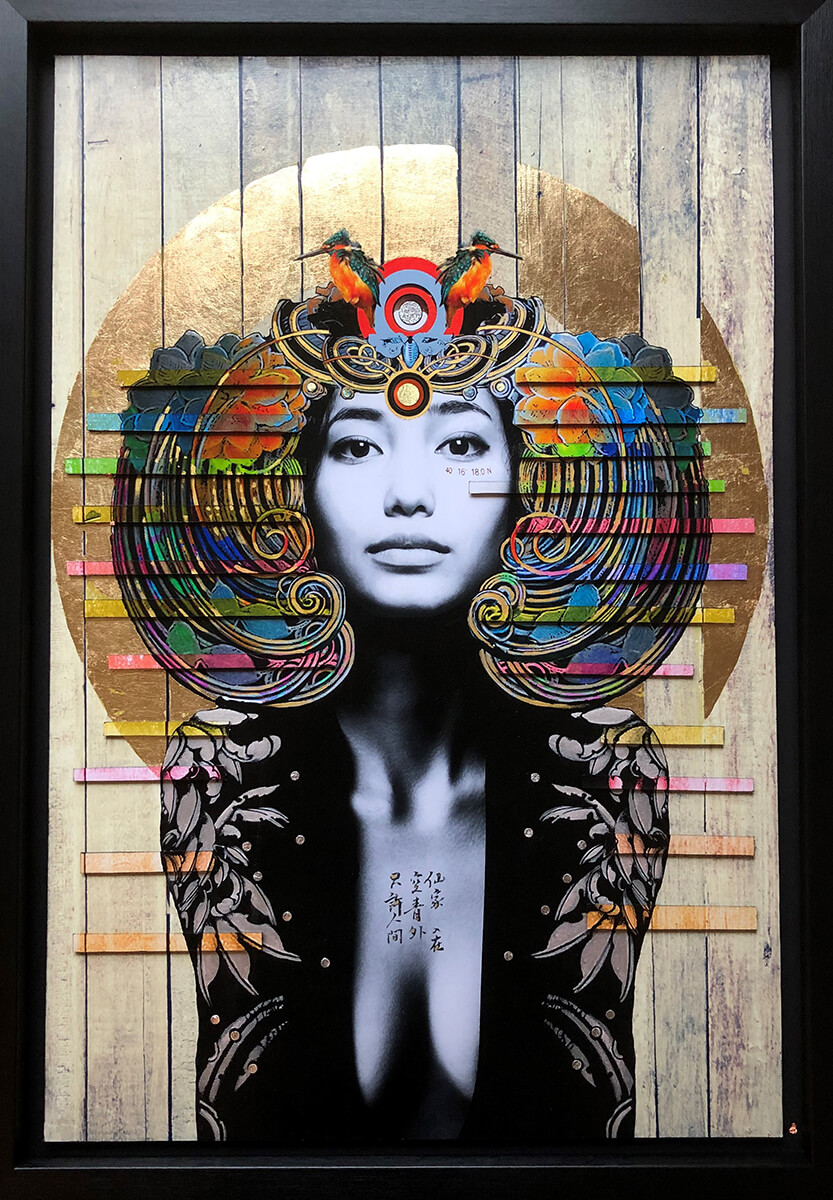The digital artwork depicts an Asian woman in a black robe with floral designs on the sleeves, leaning forward. Her robe is open, revealing her cleavage, which is adorned with Chinese characters. The background is comprised of wooden panels with gold foil painted in a circular halo shape. Within this golden circle, a vibrant swirl of colors—orange, blue, green, yellow, and pink—creates the effect of a bob hairstyle. At the center top of this colorful swirl, two orange birds face opposite directions, resting on her head like a crown. The woman's skin is rendered in black and white, contrasting with the bold, colorful elements surrounding her. Additionally, she has tattoos on her chest and under her eye. This modern, visually striking piece of wall decor combines the monochromatic photograph with lively digital artwork, creating a unique and captivating composition.